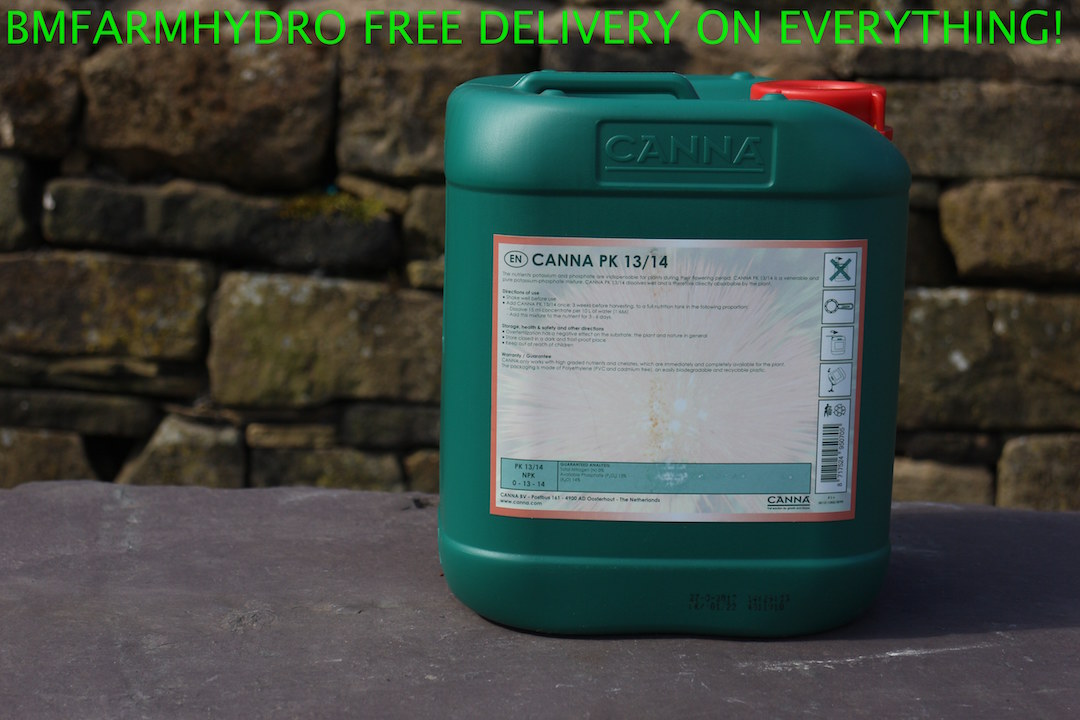The image features a green plastic canister, resembling a gas can, with a prominent red nozzle and a black cap. The label on the canister reads "Canna PK 13/14," which appears to be the product name with green writing. The canister is positioned on a table in front of a stone wall. On the stone wall, there is green text that reads "BM FARM Hydro Free Delivery on Everything!" Additionally, there are several small notices on the canister's label, including images such as one with an "X" and other symbols related to usage instructions and safety warnings.